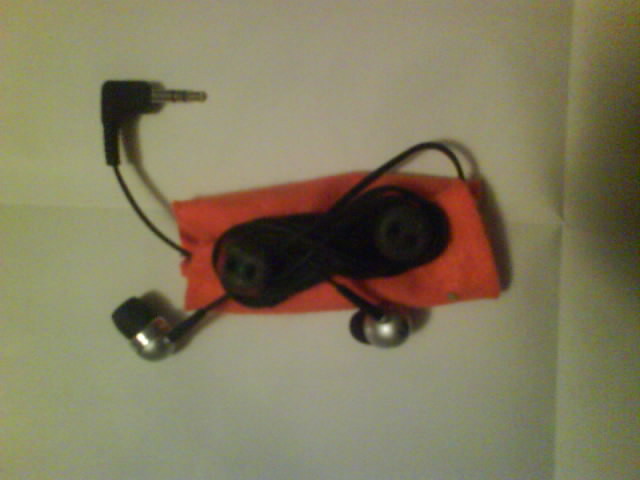The photograph showcases a pair of earbuds laid out on a coral-colored soft carrying case, which appears to be made of fabric. The earbuds are silver with black cushions and have a thin black wire that is neatly bundled together. The wire leads to a black audio plug with a metallic tip, protruding from the left side of the carrying case. The background is a beige piece of paper with visible crease lines, suggesting it has been folded into fourths. The vertical crease runs close to the right edge of the image while the horizontal crease intersects near the middle. The overall image is somewhat out-of-focus and blurry, adding a sense of softness to the scene.